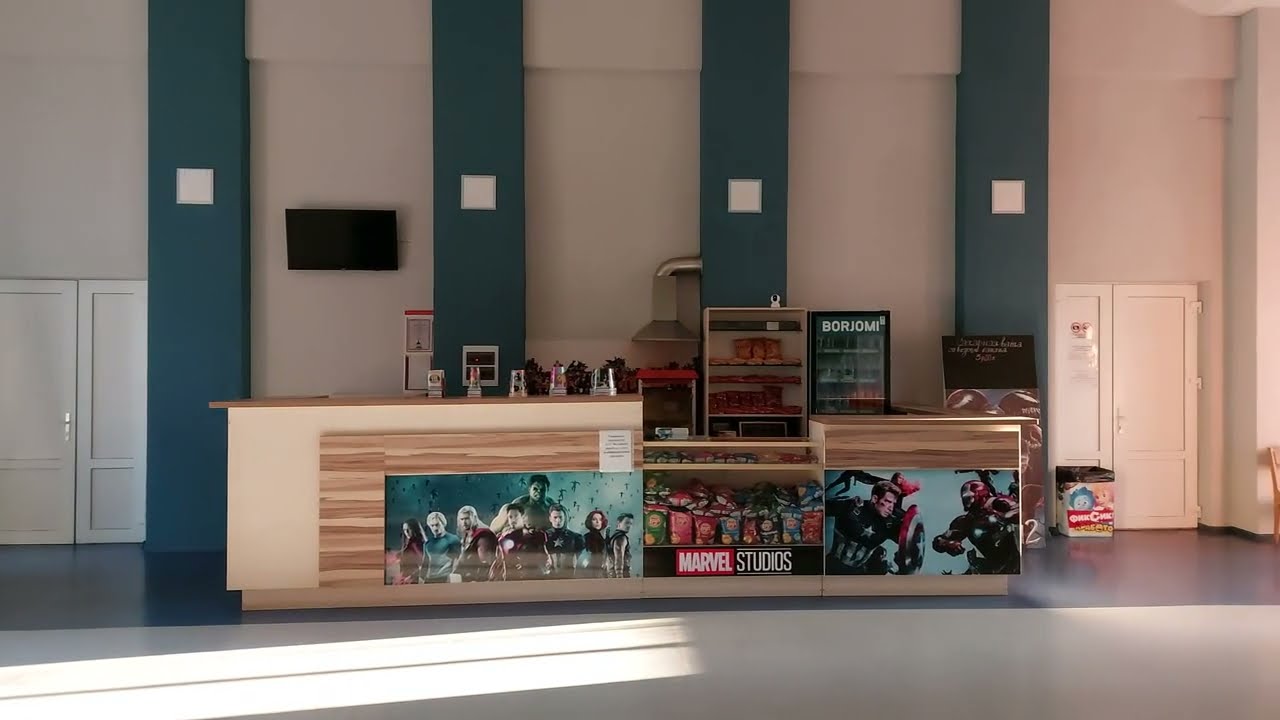The image depicts an empty concession stand inside a movie theater. Prominent movie posters line the front of the beige rectangular wooden stand, with notable titles from Marvel Studios featuring Captain America and the Avengers. The stand displays a variety of snacks, including chips and candies, and behind it, there are cabinets stocked with cold beverages and possibly a popcorn machine with red packaging. The wall behind the stand is adorned with four tall rectangular blue columns, accentuating the movie-themed decor. The clearly visible white doors on either side of the image likely lead into the actual theater halls. The floor features a white and blue pattern, and shafts of light illuminate the area, adding to the brightly lit, yet unoccupied, atmosphere. The overall impression is that the photo was taken during a time when the theater was not in operation, possibly during the COVID-19 pandemic.